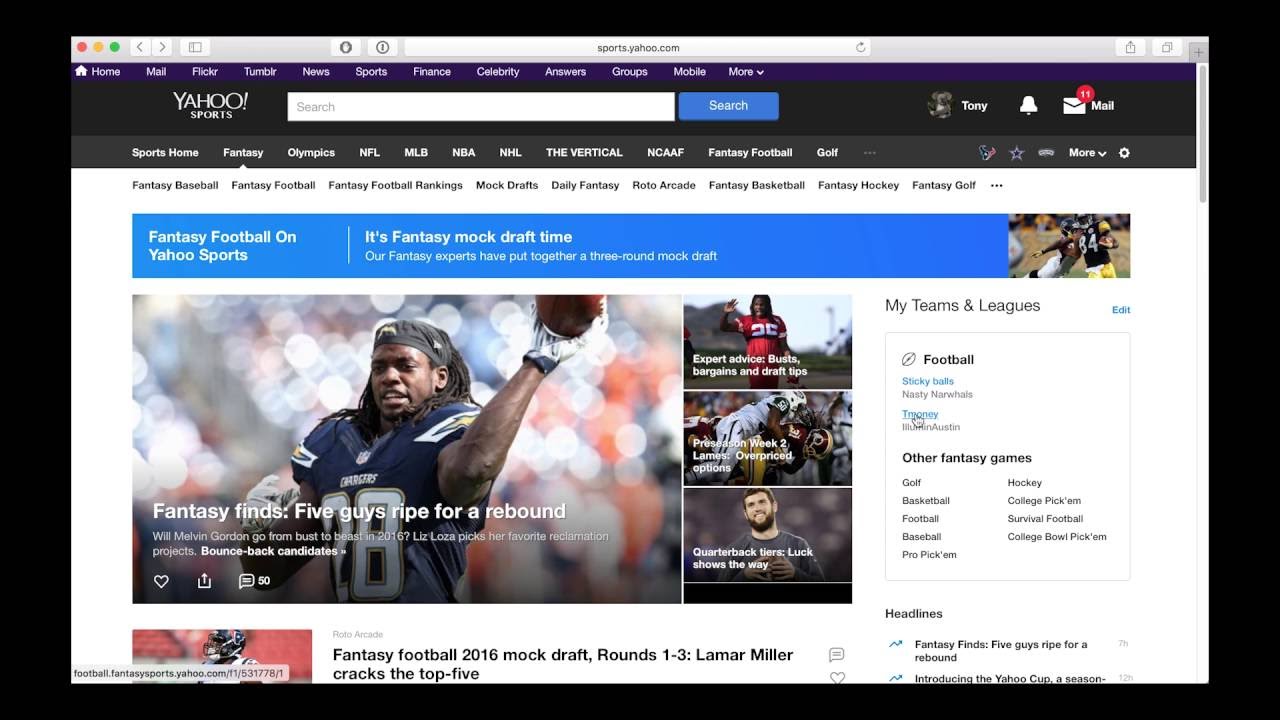Here is a cleaned-up and detailed caption for the described image:

---

This image captures an intricate view of a Yahoo Sports webpage on a computer screen. The interface is surrounded by a black frame, indicating that this is not a black-and-white image but rather the distinctive dark mode of the site. In the top left corner of the screen, standard MacOS navigation dots—red, yellow, and green—are visible, along with left and right arrows and an unidentified symbol. The user's browser is currently open to "sports.yahoo.com."

At the top of the page, a series of navigation options are presented: Home, Mail, Clicker, Tumblr, News, Sports, Finance, Celebrity, Answers, Groups, Mobile, and More. Directly below this, the header announces "Yahoo Sports" with a logo and a search bar. The user, identified as Tony, displays a close-up avatar of his face next to his name. The notification icon shows no new alerts, but Tony has 11 unread emails.

Further down, the webpage provides an array of sports categories: Sports Home, Fantasy, Olympics, NFL, MLB, NBA, NHL, The Vertical, NCAAF, Fantasy Football, and Golf. There is also a 'Star' icon for favorites and additional settings on the right.

The focal content of the screen indicates that Tony has selected Fantasy Football. The subcategories listed are Fantasy Baseball, Fantasy Football, Fantasy Football Rivals, Mock Drafts, Daily Fantasy, Roto Arcade, Fantasy Basketball, Fantasy Hockey, and Fantasy Rock. The blue header bar states "Fantasy Football on Yahoo Sports." The featured article begins with "It's Fantasy Mock Draft time. Our fantasy experts have put together a three-round mock draft," accompanied by an image of a player diving towards a Steelers player in possession of the ball.

An adjacent advertisement labeled "Fantasy Ponds" promotes various fantasy football topics such as Melvin Gordon’s transformation from bust to beast in 2016, as highlighted by Liz Loza. The right side of the page displays expert advice categories with corresponding images, including a Kansas City Chiefs player, under headers like "Bust, Bargain, and Draft Tips" and "Preseason: Lane’s Overpriced Options," featuring athletes from Washington Redskins and Green Bay Packers.

The bottom right section includes a breakdown of quarterback tiers, with Andrew Luck prominently mentioned as leading the way. Just below, there’s a section titled "My Teams and Leagues" with an edit button, featuring user-generated team names such as Sticky Balls, Nasty Narwhals, and Timoney. Other fantasy games listed include Golf, Hockey, Basketball, College Pick'em, Football Survival, Baseball, and Pro Pick'em.

The screen captures the top portion of the "Fantasy Football 2016 Mock Draft" article, which reveals the top 5 picks of the first three rounds. Additionally, it showcases headlines like "Fantasy 5," with further insights and top-tier recommendations from five fantasy sports experts.

---

This caption provides a comprehensive and detailed description of the Yahoo Sports webpage as captured in the image.